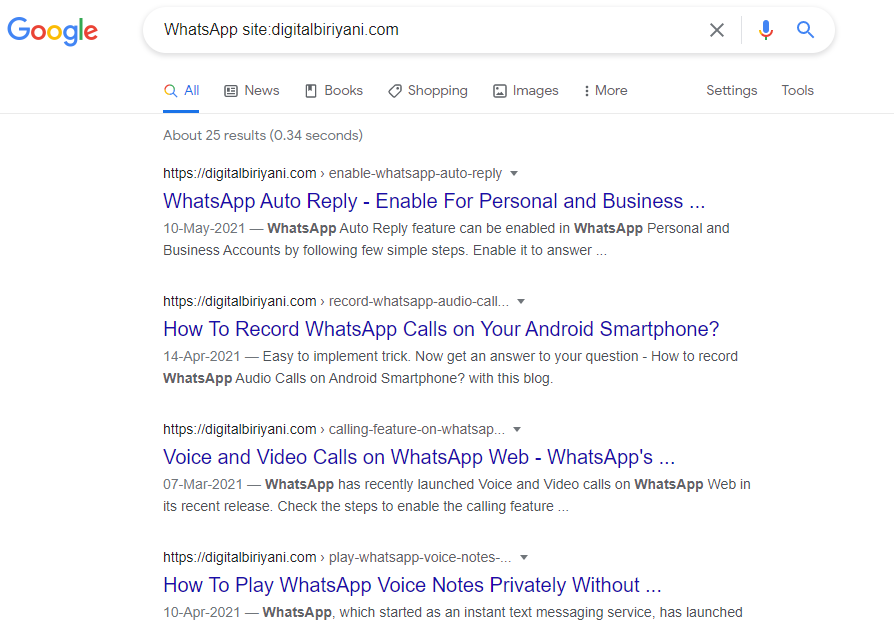This is a detailed screenshot of a Google search results page for the query "WhatsApp site: digitalbiriani.com." The search results display several entries linking to articles on the DigitalBiriani website, each providing informative content about various WhatsApp features and functionalities. 

1. The first result is titled "WhatsApp Auto-Reply Enable for Personal and Business." The summary highlights that WhatsApp auto-reply can be enabled for both personal and business accounts by following a few simple steps. This feature allows automatic responses to be sent.

2. The second result is "How to Record WhatsApp Calls on Your Android Smartphone." This entry details an easy-to-implement trick to answer the user's query about recording WhatsApp audio calls on an Android device.

3. The third result is "Voice and Video Calls on WhatsApp Web." This article discusses WhatsApp's recent release that enables voice and video calls on WhatsApp Web, along with the steps to activate these calling features.

4. Lastly, "How to Play WhatsApp Voice Notes Privately" discusses a feature of WhatsApp, which started as an instant text messaging service. The article elaborates on how to play voice notes privately.

The entire screenshot is neatly captured in a rectangular shape, providing a clear view of the search results and the brief descriptions of each linked article.